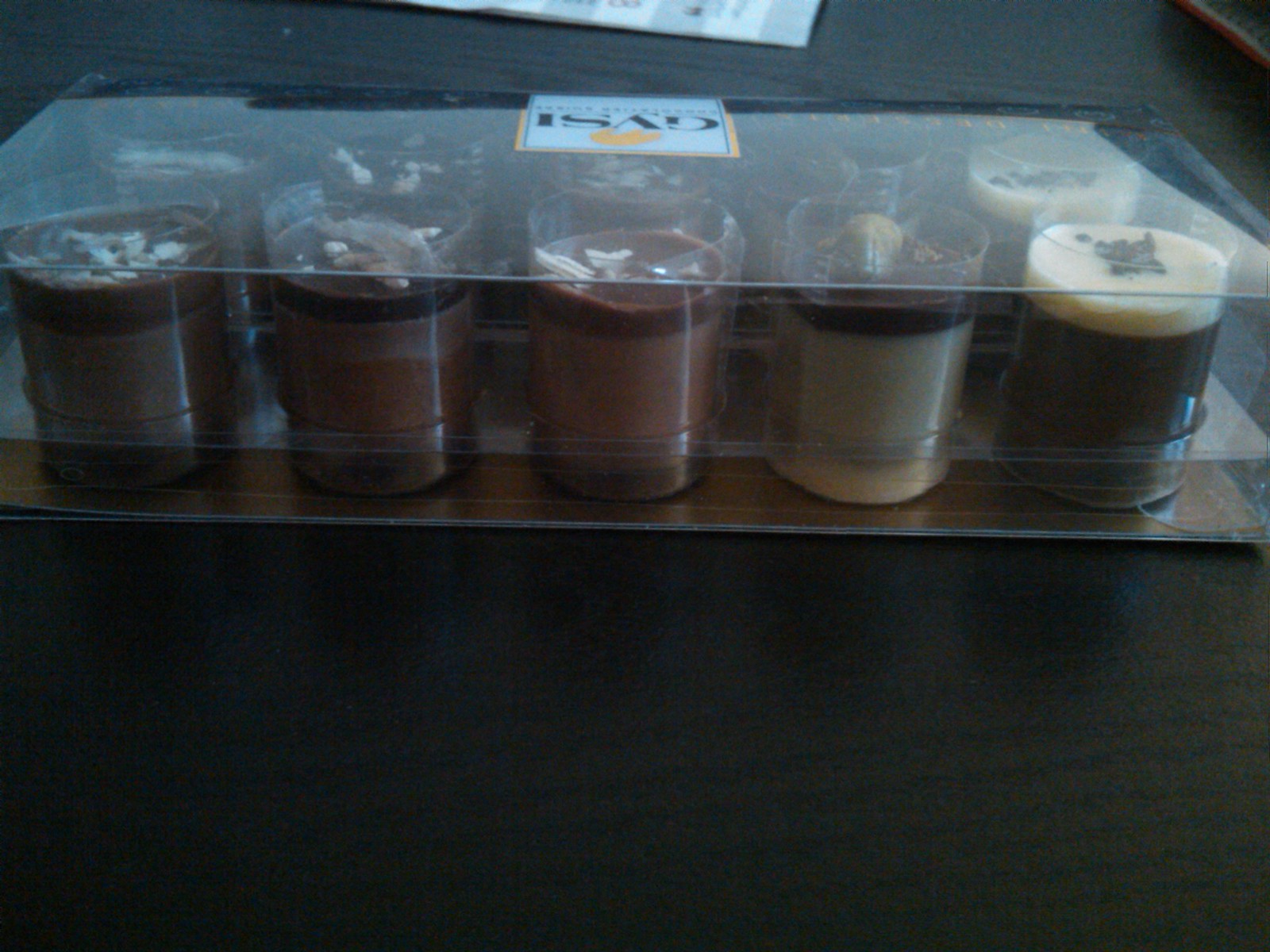The image showcases a close-up of a see-through plastic package containing ten cylindrical dessert-style pudding cups, arranged in two rows of five. Each dessert cup appears to be of a slightly different flavor or design, featuring layers in various shades of tan, brown, dark brown, and even some green to yellow gradient. These layers are topped with various decorations, such as white dots and fragments, enhancing their visual appeal. The rigid plastic packaging has a sturdy base designed to prevent the cups from moving around. Although the plastic container is entirely transparent, it features a white label in the center of the back, with bold black letters "GVSI" printed in a thin outline. The entire package is situated on a dark wooden surface with discernible grain, adding a textured background to the tightly cropped image. The edges of the package are slightly cut off, and the bottom left corner appears almost black due to poor lighting.